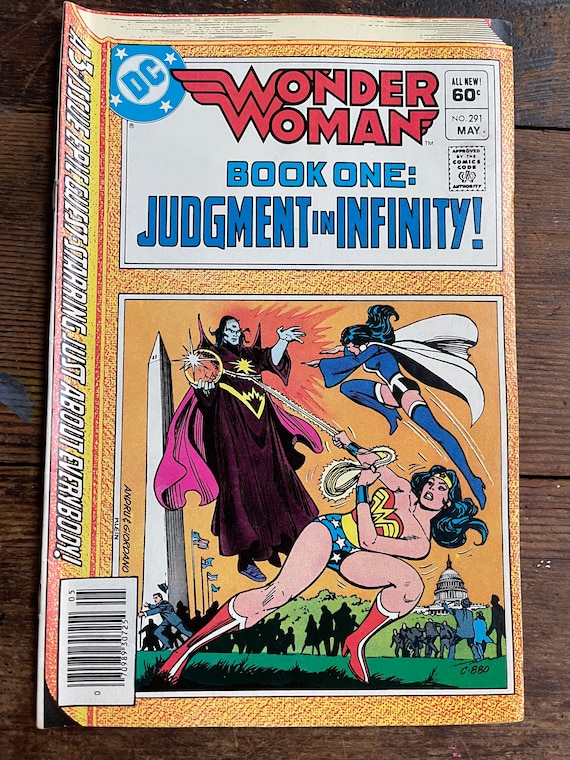This vertically-oriented, rectangular image depicts a well-worn comic book titled "Wonder Woman." The comic has a prominent binding, indicating it’s rather thick, and a barcode partially extending from the spine to the front cover, suggesting it might be a paperback. The title "Wonder Woman" is boldly printed in red, block letters outlined in black at the top of the cover. Below that, in blue letters, it reads "Book One: Judgment in Infinity." The cover features a circular DC logo with four stars on the upper left side and a white square border at the bottom encasing an action scene illustration.

The central image on the cover showcases Wonder Woman, donned in her iconic swimsuit attire and red boots, pulling a rope with her golden lasso that ensnares a villain dressed in a purple robe and cape. Wonder Woman is engaged in dynamic motion, lunging and turning as she overpowers her enemy. The background includes a field with a monument on the left and people fleeing in the backdrop. The wooden platform the comic rests on can be seen, brown in color with distinct lines running across it.